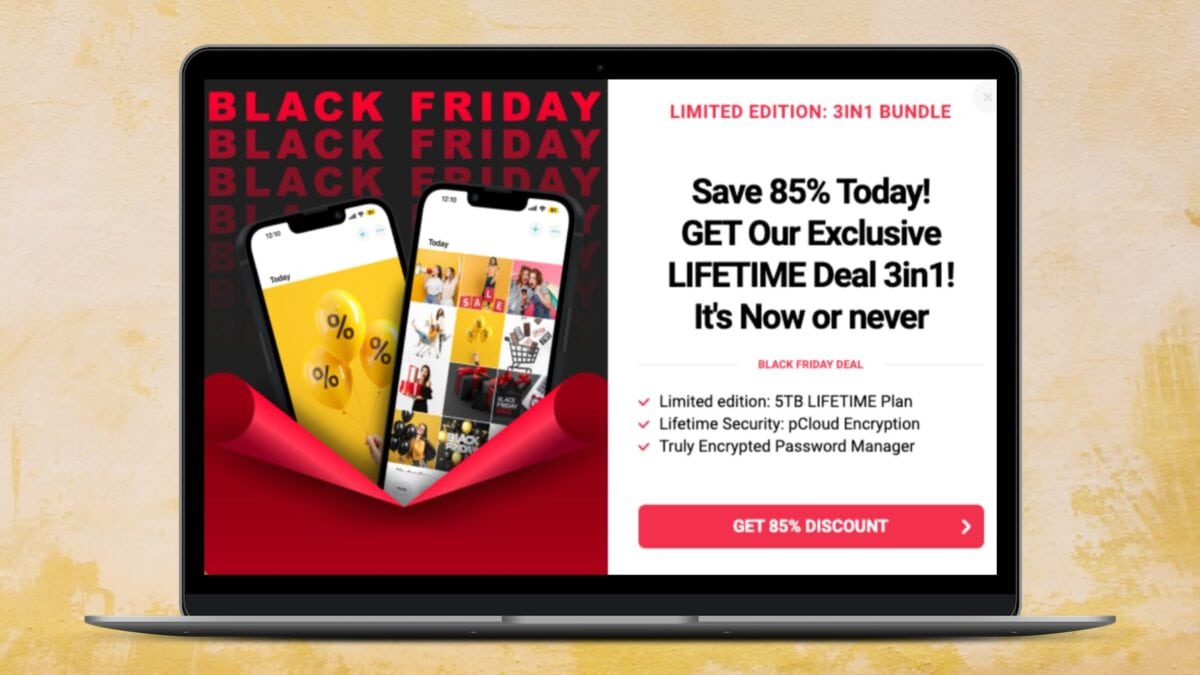The advertisement features a visually striking and animated depiction of a Black Friday sale. The design centers around a large tablet screen set on its side on a small grey shelf, against a soothing blend of pale yellow and pale peach background. The tablet itself is outlined in a bold black for emphasis. 

The tablet's display is smartly divided into two vertical sections. 
- The left section features a dynamic animation where the words "Black Friday" are prominently displayed in vivid red at the top, with the text gradually fading down the section repeating "Black Friday" in a fading sequence. 
- Below, two vertical cell phones are showcased, appearing as if they are emerging from behind a torn red piece of paper, enhancing the sense of urgency and excitement.

The right section is rich with bold text information in contrasting colors:
- At the top in bright red, it announces a "Limited Edition 3-in-1 Bundle."
- Following this in deep black text are compelling offers: "Save 85% today, get our exclusive lifetime deal 3-in-1. It's now or never."
- Further down, in red again, it reiterates the "Black Friday deal."
- Below that, more details are provided, culminating in a red bar that commands attention with an enticing call-to-action: "Get 85% discount," prompting users to click through for the offer.

The carefully structured design and color palette effectively highlight the urgency and exclusivity of the Black Friday deals, encouraging immediate action.